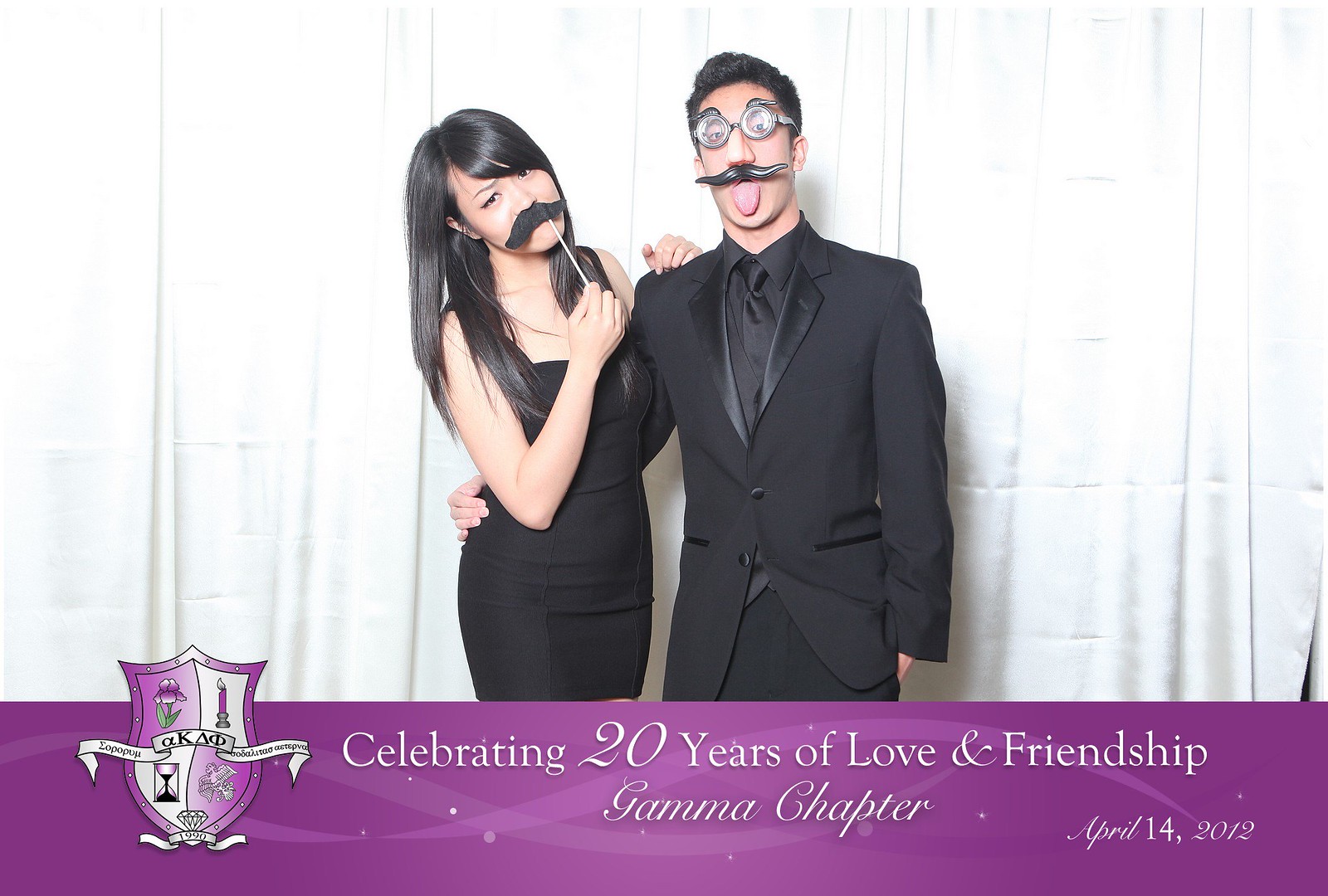This photograph, likely taken in a photo booth at a formal event, features a playful Asian couple dressed in black attire. The man is on the right, sporting a black tuxedo, black shirt, and black tie along with cartoonish round glasses, a fake nose, and a fake black curly mustache. The woman on the left has long black hair with side-swept bangs, is dressed in a sleeveless black cocktail dress, and is holding a stick-attached mustache under her nose. Both of them are posing in front of a white curtain. The bottom of the image features a purple ribbon banner with white serif font text reading "Celebrating 20 Years of Love and Friendship, Gamma Chapter, April 14th, 2012." On the left side of this ribbon is the Gamma Chapter’s shield, which is divided into four panels with distinct objects and features a white scroll across it.